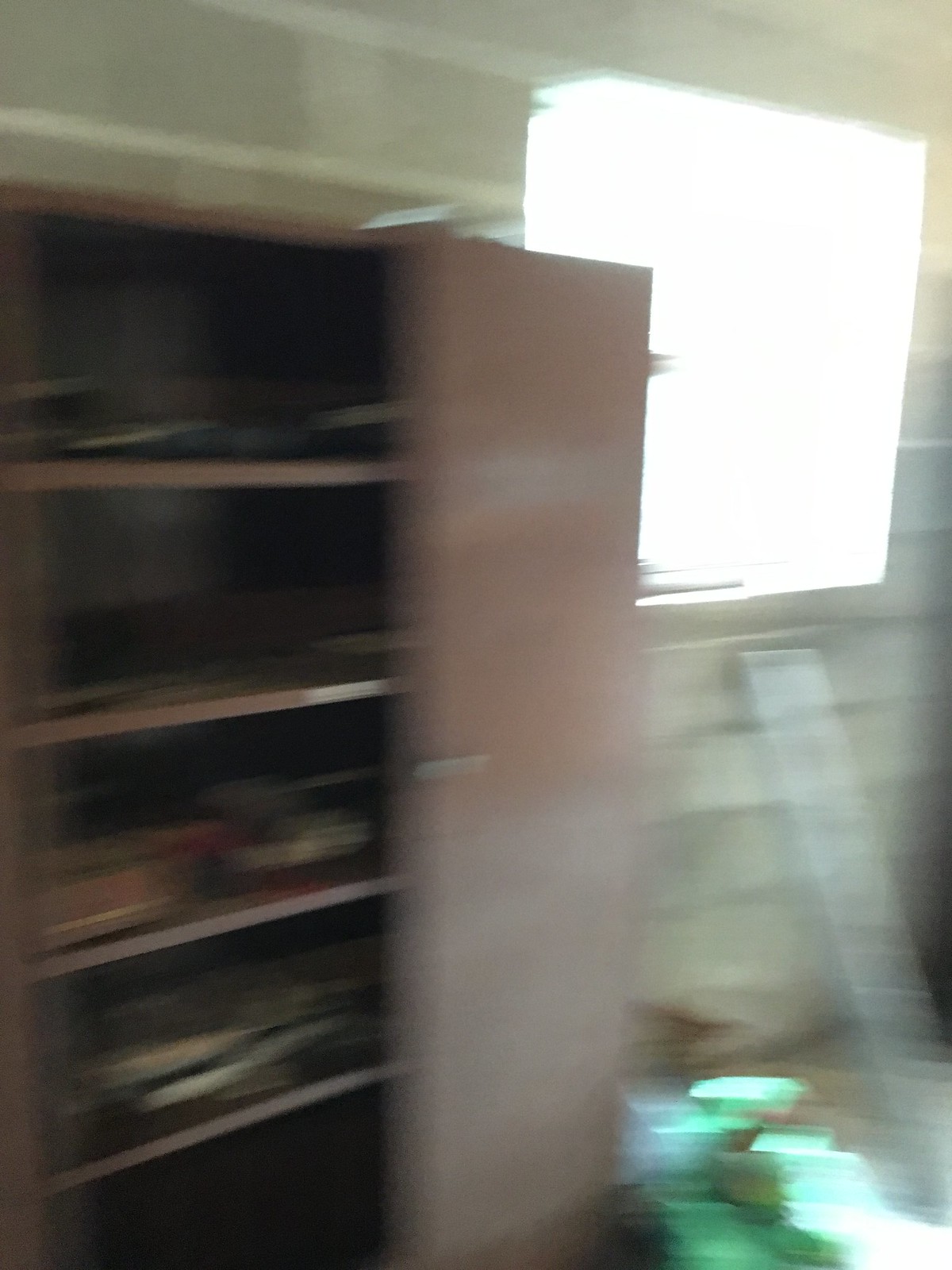In this heavily blurred image, we find ourselves in a basement setting dominated by an unfinished wall made of cinder blocks. A rectangular object is propped up under a simple hole serving as a window, hinting at the space being part of an ongoing construction—possibly a cement house still in progress. 

Against the wall stands a tan-colored cabinet with a sliding door that is partially open, revealing its contents. Reflecting the scant light, the door appears almost shut. The cabinet hosts four shelves laden with various items, adding a cluttered but homey feel. Among the items are a collection of pots, pans, and dishes, with noteworthy red shelving that holds red objects, further contributing a pop of color to the scene. Some white bowls are also visible; they appear to have handles, although this could be an illusion caused by the image's blurring.

In front of the cabinet, green Tupperware containers are scattered on the ground. A conspicuous brown stain mars the cinder block wall above, indicating either old spills or possible water damage. The overall scene paints a picture of a utility space or storage area amidst a broader home construction or renovation project.